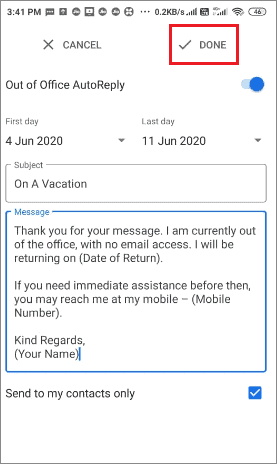**Caption:**

This image is a screenshot taken from a cell phone at 3:41 p.m., as indicated by the clock in the status bar. The battery is at 46%, and the phone interface is characterized by a plain white background with dark gray text. 

At the top of the web page, there is a toolbar displaying the word "Cancel" with an "X" icon to its left on the upper left-hand side. On the opposite side, the word "Done" appears with a checkmark next to it, both highlighted by a red rectangle that seems to have been drawn manually. 

Below the toolbar, the heading "Out of Office Auto Reply" is shown, indicating that this is a settings page for configuring an out-of-office email auto-reply. The auto-reply feature is toggled on, as evidenced by a circular toggle switch positioned to the right.

Further down, the body of the page provides the specific dates for the auto-reply:
- **First Day:** June 4, 2020
- **Last Day:** June 11, 2020

The subject of the auto-reply is simply, "On a vacation."

This screenshot essentially represents an email settings page where an individual has set up an automatic vacation response to notify senders of their absence between the specified dates.